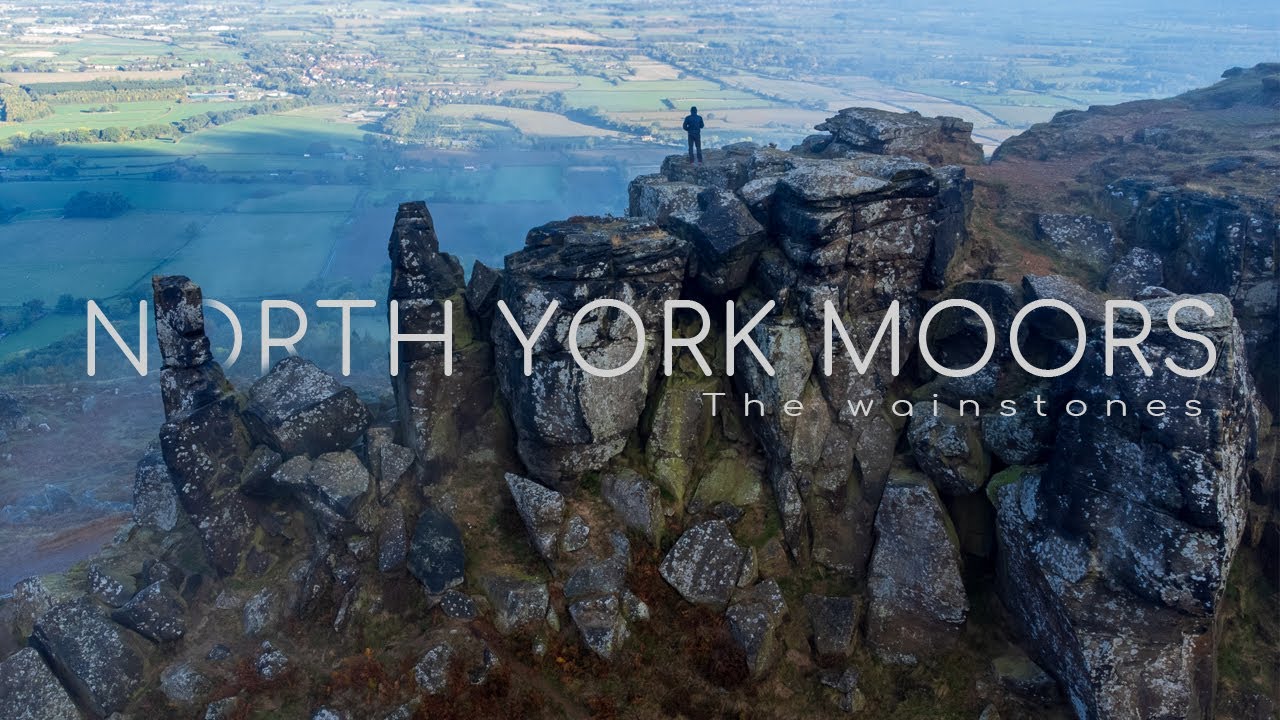The image captures an awe-inspiring view of the North York Moors, with elegantly styled white text across the middle that reads "North York Moors" in larger font and "The Wainstones" in a slightly smaller font beneath it. Dominating the foreground is a massive, rugged rock formation, the Wainstones, stretching across the bottom and middle sections of the picture. Perched atop this imposing cliff is a solitary figure, his back to the viewer, dressed in black pants and a black leather coat, hands tucked into his pockets as he gazes out. Beyond him unfolds a vast, verdant landscape of grassy fields interspersed with trees and farmland. In the background, hints of blue and white sky break through the fog, adding depth and serenity to the scene, while a small village or city peeks out from the left center of the image. This stunning photograph, potentially an advertisement, perfectly captures the dramatic beauty and scale of the North York Moors and the serene solitude of the Wainstones.